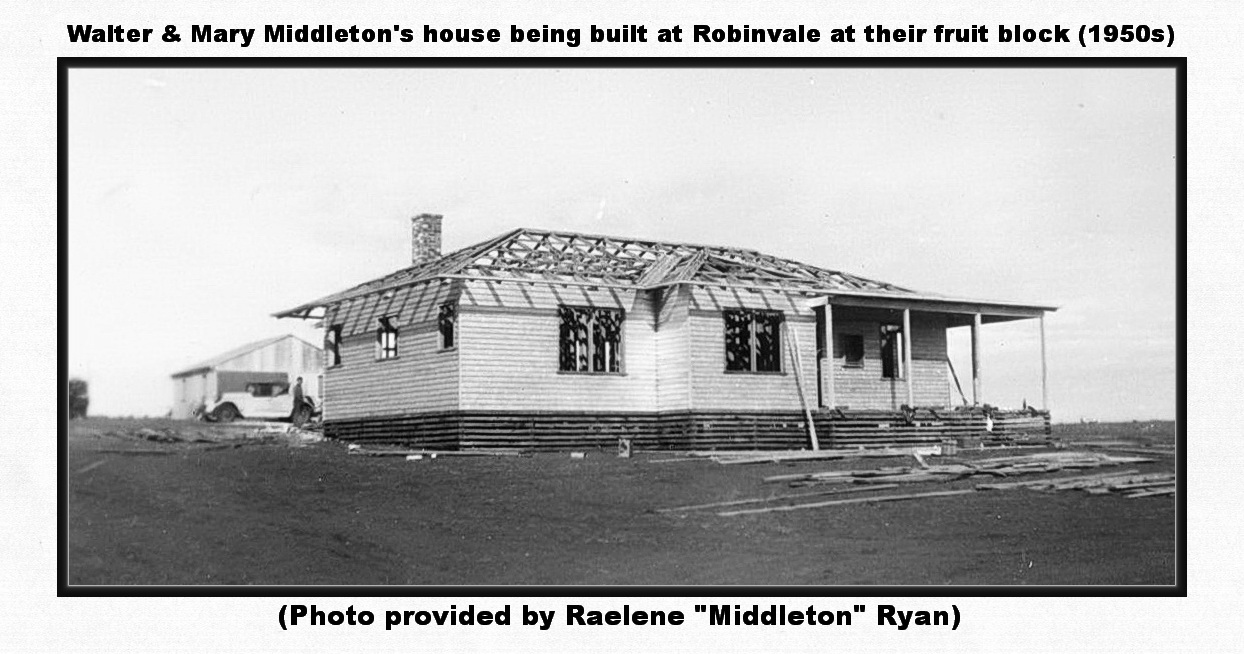This black-and-white photograph from the 1950s shows the partially constructed house of Walter and Mary Middleton, located at their fruit block in Robinvale. The house stands on a dirt plot and features a predominantly white brick exterior with a lower portion of dark bricks extending a couple of feet up from the ground. While most of the house appears complete, the roof is notably unfinished, lacking shingles. Behind the house, a vehicle is visible with a man standing beside it, possibly near a small shed or garage. The image is clear and includes a caption at the top stating, "Walter and Mary Middleton's house being built at Robinvale at their fruit block (1950s)," and a note at the bottom indicating, "photo provided by Raylene Middleton Ryan." No other objects are noticeable in the image aside from some construction materials scattered around the site.